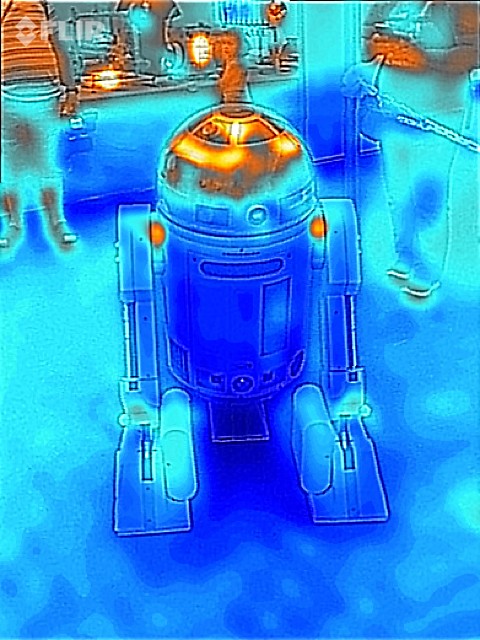The image depicts a digitally altered photograph with multi-colored effects, primarily featuring blue hues with splotches of gold. The scene is set inside a store, where various elements have been transformed by what appears to be a color temperature filter. This filter makes the ground and the robot R2-D2 from Star Wars appear blue, while the top of R2-D2's head is oddly gold or orange. In the center of the image stands R2-D2, and at the counter behind him is a little child. Also visible in the store are two adults facing the camera; one is standing, and the other, presumably a woman carrying a purse, is holding up a phone. The surreal color effects suggest an intent to visually represent temperature variations across the scene, with clothes appearing bluish and human bodies exhibiting a reddish hue.